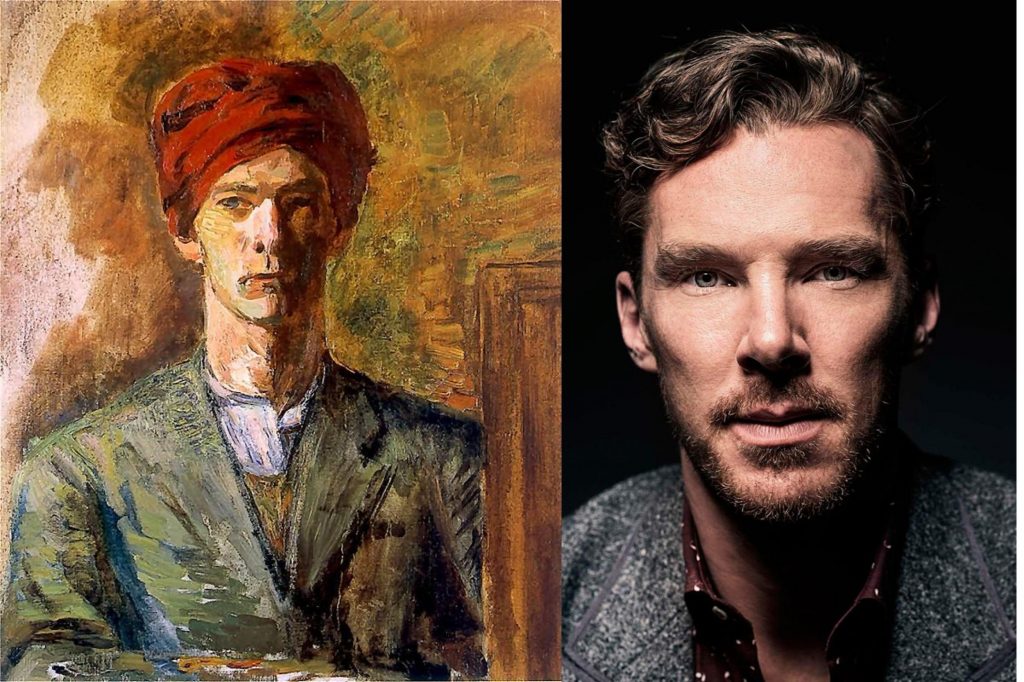The image is a horizontally rectangular, professionally staged composition divided into two distinct parts. On the right side, there is a photograph of the actor Benedict Cumberbatch. He is partially in shade and gazes directly at the viewer. Cumberbatch has a neatly trimmed goatee, curly brown hair, green eyes, and wears a grey suit over a shirt with a collar. On the left side, there is a painting of a man strikingly similar to Cumberbatch. This man, without facial hair, dons a red turban and a green jacket over a layered outfit that includes a white shirt. The background of the painting features yellow, brown, white, and green splotches applied in broad, impressionistic strokes. The stark contrast and parallel positioning of the two portraits create a visually compelling comparison between the photograph of the actor and the artistic representation of the similar looking man in the painting.